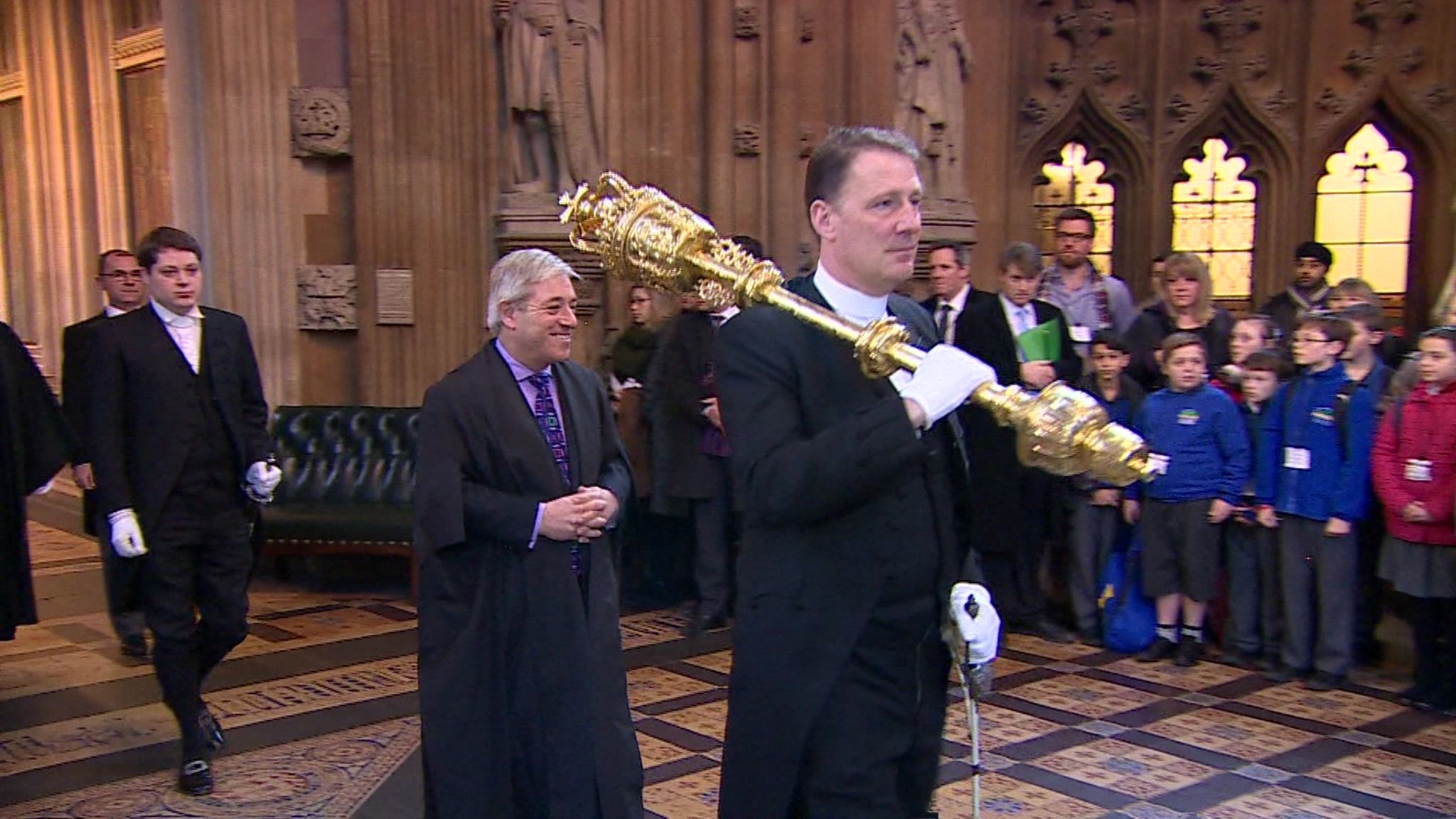The image depicts a royal proceeding set in an ornate and medieval-style hall, which might be a church or an old courthouse in a European country, possibly the UK. At the center of the procession is a Caucasian man in a black suit, wearing white gloves, and holding a large gold scepter crowned with a decorative crown at the top. Behind him, there is a second man who is also Caucasian, smiling, and dressed in a black long coat with a purple shirt and blue tie. Further behind are three more people in similar black attire. The hall is filled with a crowd, including several children in blue and pinkish-red clothing, likely accompanied by their parents. The intricate details of the setting, with its antique and ceremonial ambiance, emphasize the formality and historical significance of the event.